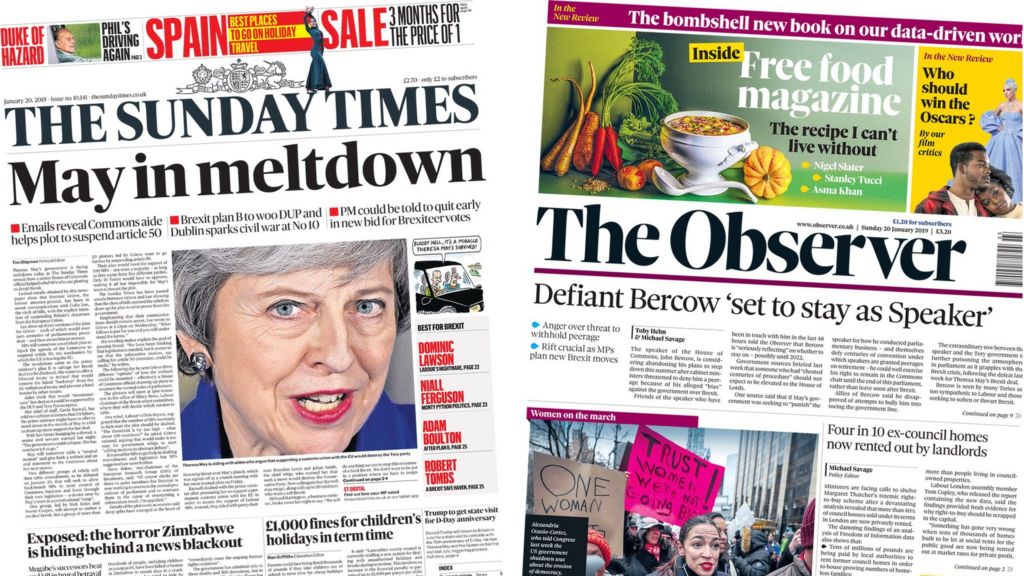This image showcases a spread from two different magazines, each featuring a variety of articles and photographs. On the left side, an issue of "The Sunday Times" includes a headline that reads "May in Meltdown," accompanied by subheadings such as "Emails reveal Commons aide's Plan B to woo, dupe," "PM could be told to quit early," "Help's plot to suspend Article 50," and "Dublin sparks civil war at Number 10 in new bid for Baxter votes." The page features a prominent photograph of a woman with short grayish-black hair and red lipstick. Her expression is tense, with her mouth slightly open and eyes fixated on something out of frame, suggesting distress or confrontation.

On the right side, an issue of "The Observer" highlights the headline "Defiant Bercow set to stay as Speaker." Below this main headline is another article noting that "Four in 10 ex-council homes now rented out by landlords." This section is illustrated with a picture of demonstrators carrying signs in a protest, emphasizing the social and political undertones of the articles within the magazine. Each page provides a glimpse into contemporary political issues and social dynamics, brought to life by vivid imagery and compelling headlines.